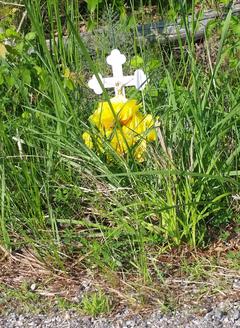This full-color, horizontally rectangular photograph captures an outdoor memorial scene during daytime. Centered in the frame, a small white cross stands prominently against a backdrop of mixed green and brown grass. The cross, adorned with decorative clover-shaped ends, marks the focal point of the image. Positioned at its base is a yellow flower, possibly plastic. Surrounding the cross, the unkempt grass and weeds grow freely, suggesting a lack of maintenance. In the upper portion of the photo lies a piece of wood, like a stick, on the ground. Adding context to the setting, a rocky area and the edge of a roadway are faintly visible in the front part of the image. The overall composition conveys a sense of solemn remembrance.